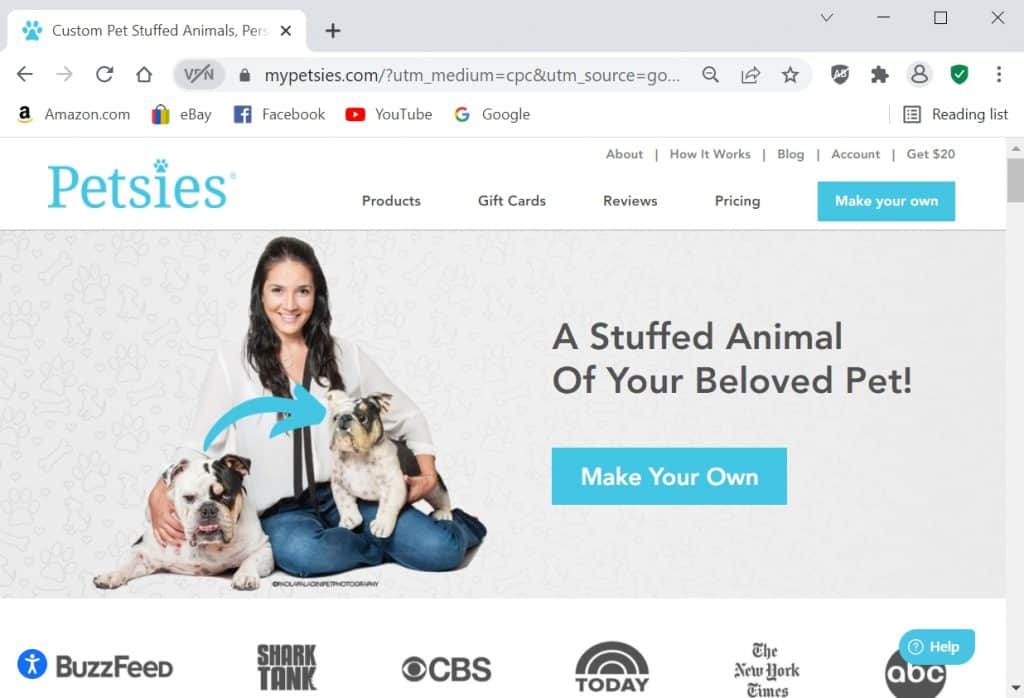The image depicts a website homepage with a focus on custom pet stuffed animals. At the top, there is a gray banner or border. Below the banner is the active webpage, featuring a small turquoise dog paw icon next to the text "Custom Pet Stuffed Animals."

Navigation icons, including a left arrow, right arrow, refresh, and home, are displayed. All icons are in darker colors except for the forward arrow, which is light gray. The website address is visible below these icons.

Scrolling down, icons for Amazon.com, eBay, Facebook, YouTube, and Google are present, suggesting integrated links or social media connections.

The background features the word "Petsies" in turquoise. Below this are navigation options: "Product," "Gift Cards," "Reviews," "Pricing," and "Make Your Own," with "Make Your Own" highlighted in a blue background with white text. Above these options are additional links, including "About," "How It Works," "Blog," "Account," and "Get $20."

An image on the webpage shows a woman sitting with her legs extended in front of her. She holds a stuffed animal under her left arm, and her real dog rests under her right arm. Text beside this image reads, "A stuffed animal of your beloved pet." The webpage also features logos for BuzzFeed, Shark Tank, CBS Today, The New York Times, and a help section.